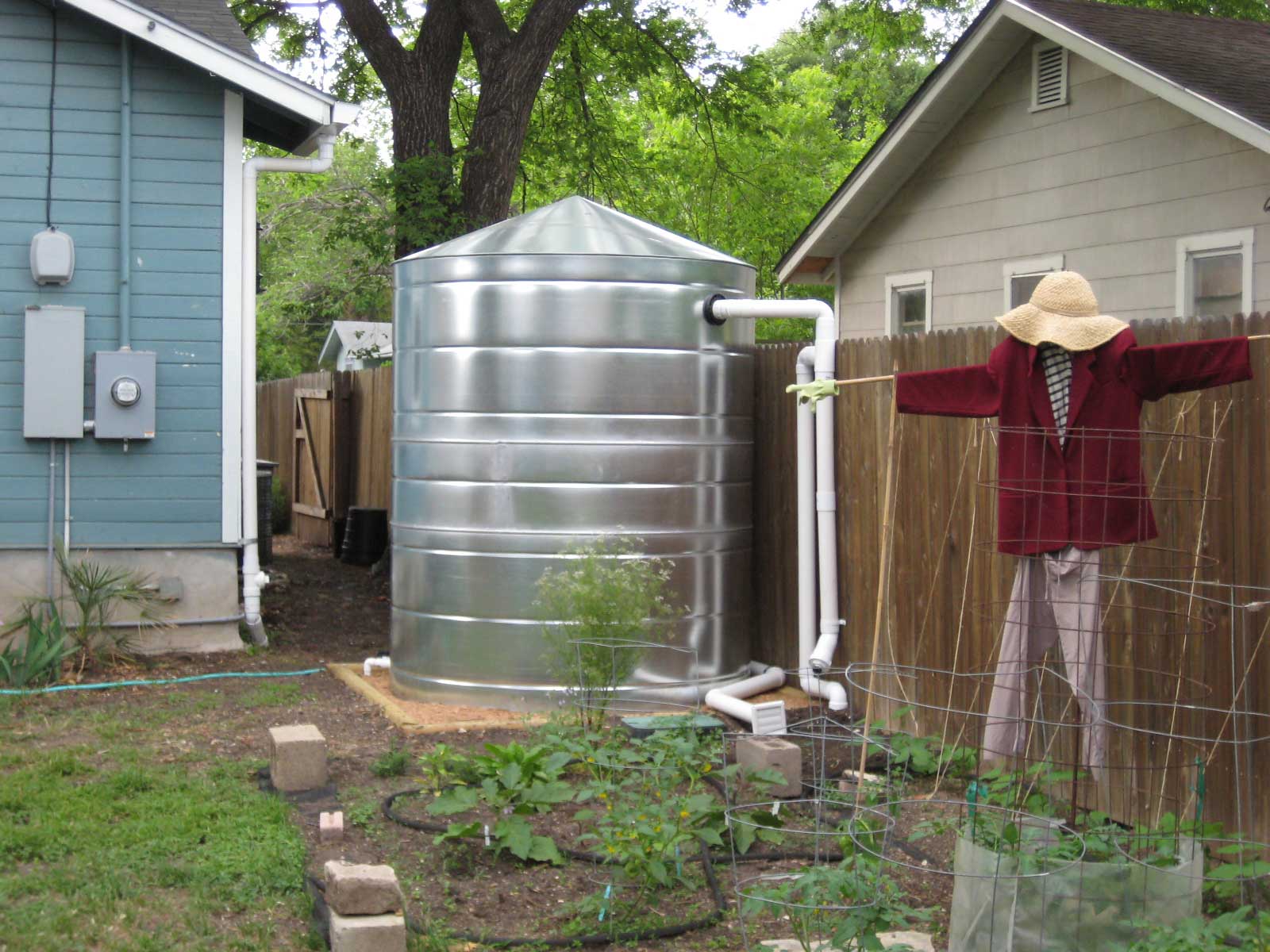The image depicts a detailed scene of a home garden in a residential backyard. Central to the garden is a large silver metal cylinder used for watering, topped with white PVC pipes that descend into the garden area. To the right of this setup is a wooden fence, and a scarecrow is positioned in front of it, adorned with a straw sun hat, a red jacket, a black and white scarf, and beige pants. The garden itself is bordered by concrete blocks and features small green plants with wire structures supporting them. In the background, you can see a tan house with white trim and a black roof, displaying three windows, and to the left, a section of a blue house with white trim and stone underpinning. The bright, white sky suggests it's daytime, and a tree is visible in the distance, completing the serene backyard scene.